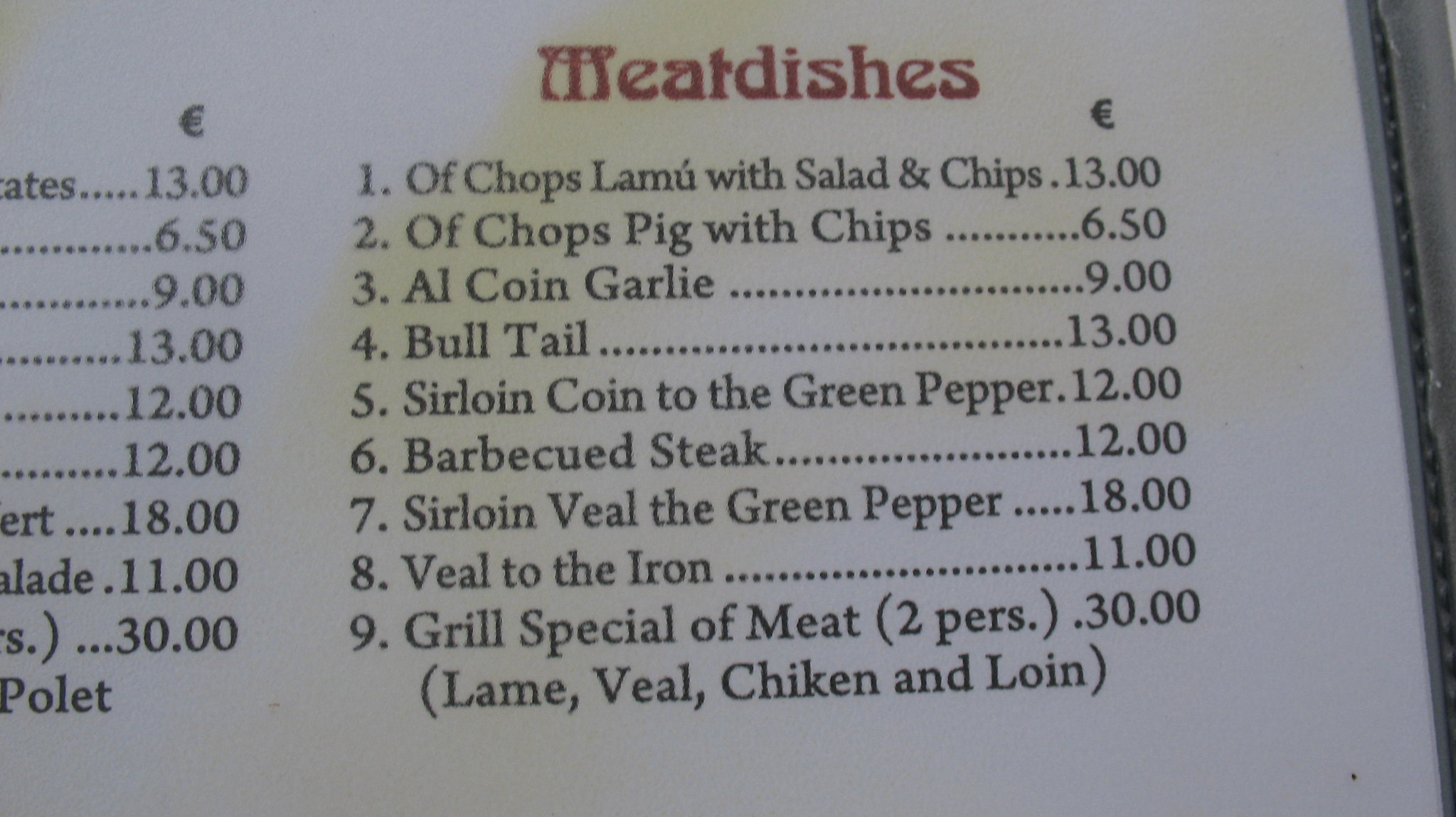This image captures a focused view of a white menu with black lettering, featuring a prominent "Meat Dishes" heading in red at the top. The menu, displaying nine distinct meat dishes and their respective prices in Euros, fills the entire frame, with only a small portion of the menu visible on the right side. The listed items include "chops lamu with salad and chips" for €13, "chops pig with chips" for €6.50, "A1 coin garlic" for €9, "bull tail" for €13, "sirloin coin to the green pepper" for €12, "barbecue steak" for €12, "sirloin veal the green pepper" for €18, "veal to the iron" for €11, and the "grilled special of meat for two persons" at €30. The description beneath the grilled special mentions a mix of lamb, veal, chicken, and loin. A second column shows prices but the corresponding items are obscured in the image.